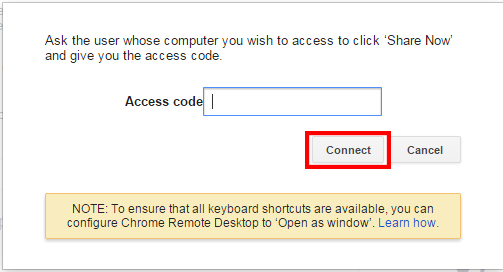This image features a user interface pop-up designed for remote desktop access on a computer. The predominantly white window displays a set of instructions in black text, which reads: "Ask the user whose computer you wish to access to click 'Share Now' and give you the access code." Directly below this instruction, there is a text box labeled "Access Code," enclosed within a blue rectangular border, indicating a field where the user can type the provided access code.

Beneath the access code input field, there are two buttons: one red button labeled "Connect" and a gray button labeled "Cancel." Both are clearly demarcated for distinct interactive choices.

At the bottom of the pop-up, a beige or yellowish rectangular box contains additional information. The text in this box states: "Note: To ensure that all keyboard shortcuts are available, you can configure Chrome Remote Desktop to open as a window," followed by "Learn How" in blue text, suggesting it is a clickable link for further instructions.